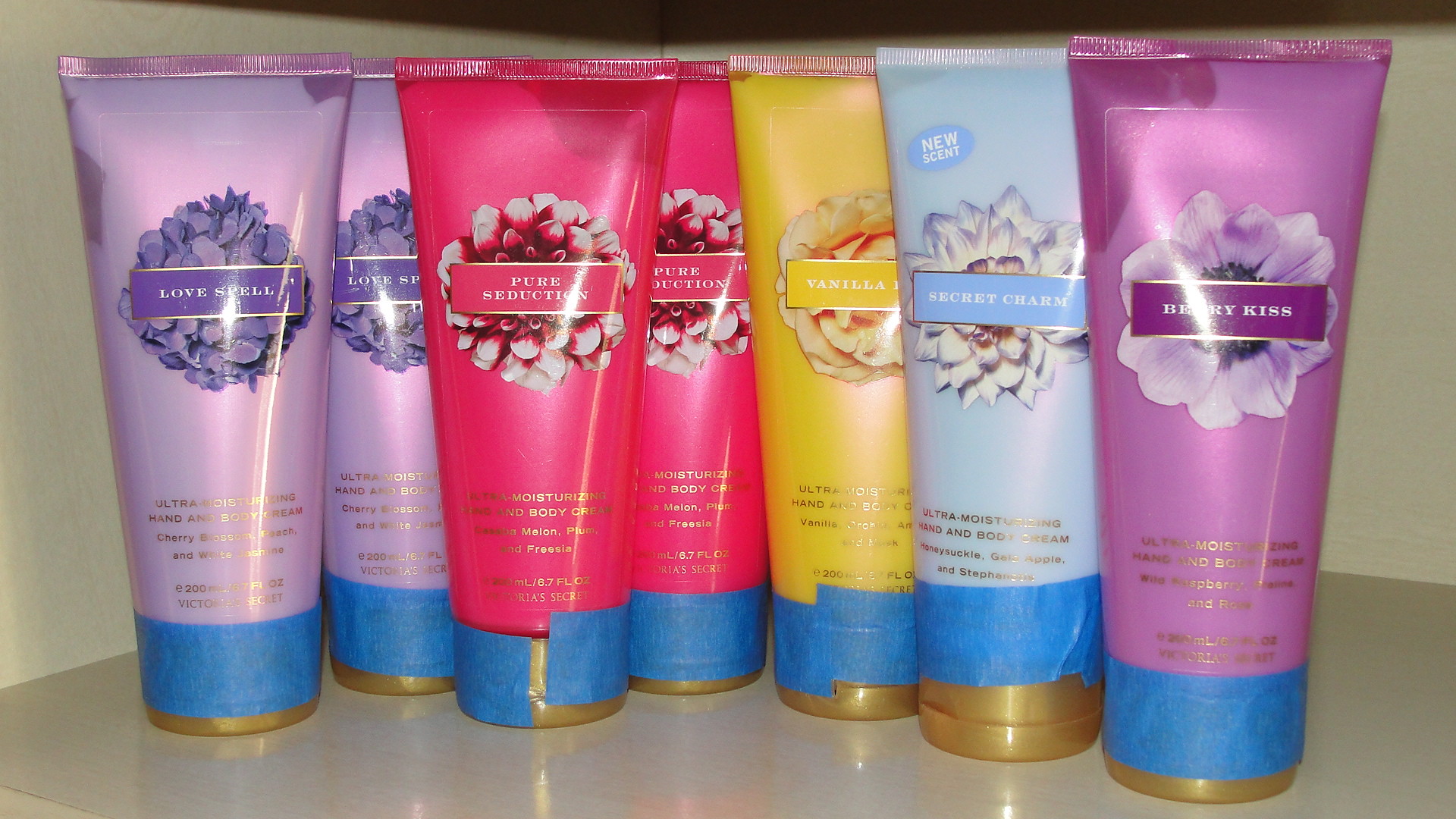This image showcases a neatly organized display of hand and body creams, each presented in vibrant, plastic tubes adorned with gold, flip-top caps. The tubes sit on an ivory shelf, likely in a store or on an e-commerce website. Blue painter's tape wraps around the base of the caps and bodies of the tubes, possibly for branding or promo purposes. The arrangement includes two lavender tubes labeled "Love Spell," two deep pink tubes marked "Pure Seduction," a yellow tube for "Vanilla," a light blue tube inscribed "Secret Charm," and a dark rose-colored tube titled "Berry Kiss." Each tube features small gold printing just above the cap and a delicate flower design on the front. One of the products is marked with a "New Scent" label.